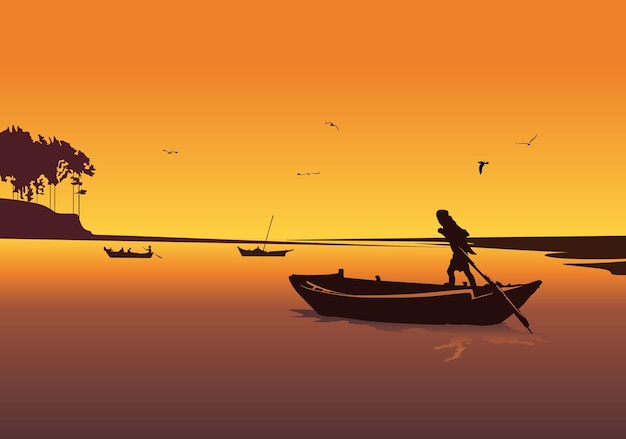This is a detailed artistic illustration of a tranquil lake at sunset, featuring rich gradients of orange and yellow hues that blend together in the sky and reflect off the water's surface. The focal point is a trio of silhouette boats—all in various stages of rowing or standing, outlined in deep purple and black against the vibrant backdrop. 

The foremost boat features a man standing, pushing the boat forward with a pointed oar that dips into the water, demonstrating a sense of motion. Farther back, two additional boats are visible; one contains a single figure holding a long stick, while the other holds multiple people—possibly three—with one individual actively rowing. 

Birds, sketched in black silhouettes, soar above the scene, adding to the serene atmosphere. On the left side of the image, a landmass resembling an island with tall trees—likely palm trees—casts a purplish-black outline, punctuating the horizon. Meanwhile, the right horizon remains flat, seamlessly disappearing into the distance, creating a sense of expansive calm. 

The composition and color palette suggest a sunset, further emphasized by the silhouettes that enhance the timeless, almost cartoony essence of the scene. There are subtle details, such as the calmness of the lake and the simplistic yet evocative portrayal of figures, which evoke an idyllic, serene setting, reminiscent of a bygone era or an idealized, peaceful moment.